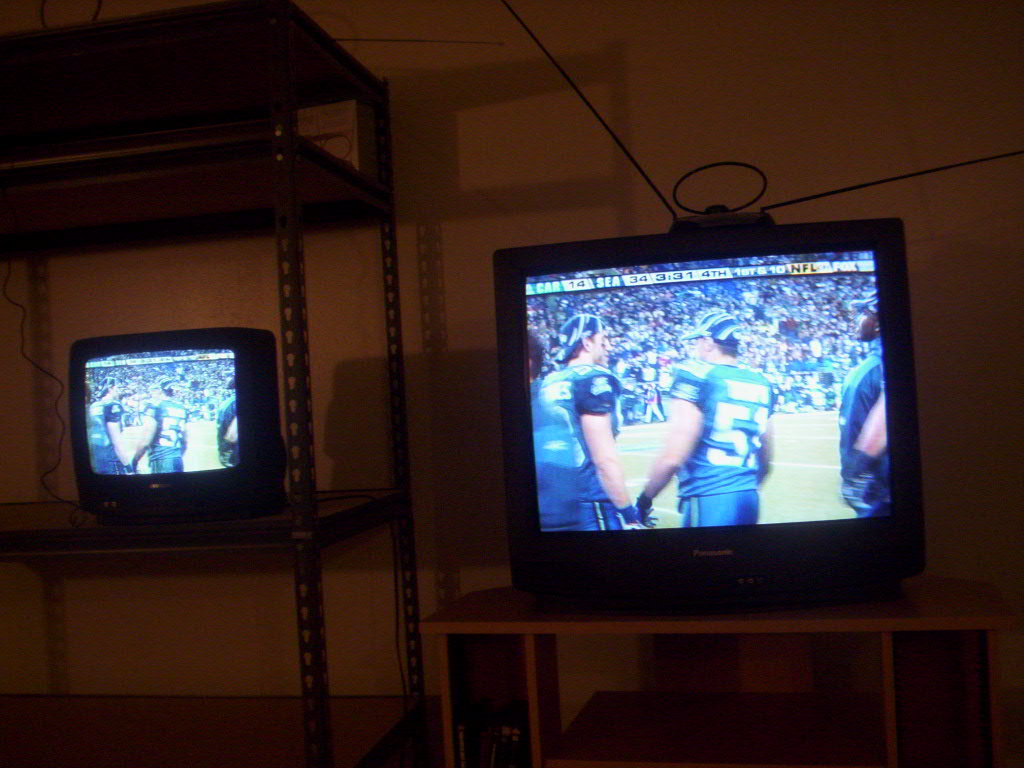In a dimly lit room, two vintage tube-style televisions are showing the same football game. The TV on the left is small and situated on the middle shelf of a wire shelving unit. This unit features multiple tiers with varying shelf spacing. The screen of the small TV isn't very vivid, displaying faint images of football players. The TV on the right is significantly larger and sits on a slender wooden TV stand. It features a set of two metal antennas and a circular antenna pointed downward, all mounted on a black base. Both TVs add an old-timey ambiance to the otherwise nondescript dark room, where the only notable background feature is the indistinct back wall. To the side of the larger TV stand, there are rectangular openings that might contain DVDs or books, although they remain dark and out of focus.